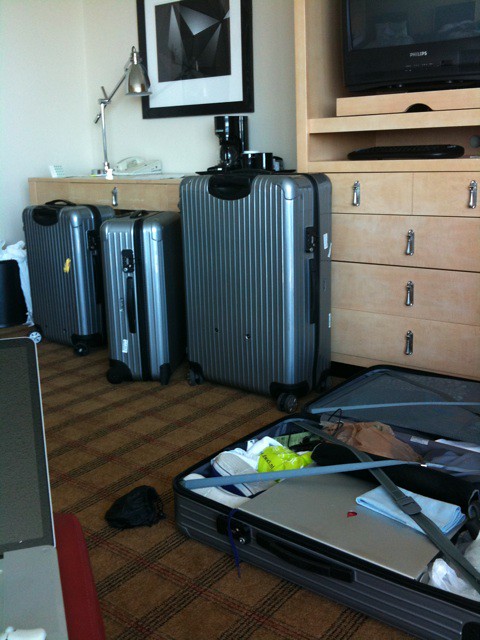The photograph captures a generic, mass-manufactured hotel room setting with a light grey or white wall adorned with an abstract black-framed artwork depicting a brownish shell design. In the right portion of the image, there's a light beige wooden cabinet topped with a TV set. Positioned below a table with a metal lamp, three metallic silver suitcases stand upright, while a fourth suitcase lies open on the brown, towel-patterned carpet floor. Inside the open suitcase, clothes, a laptop, and various objects, including a small black item, a red item, and a grey item, are visible, with security straps crossed over them to secure their placement. A black object and another unidentified black and red object rest beside the open suitcase on the floor.